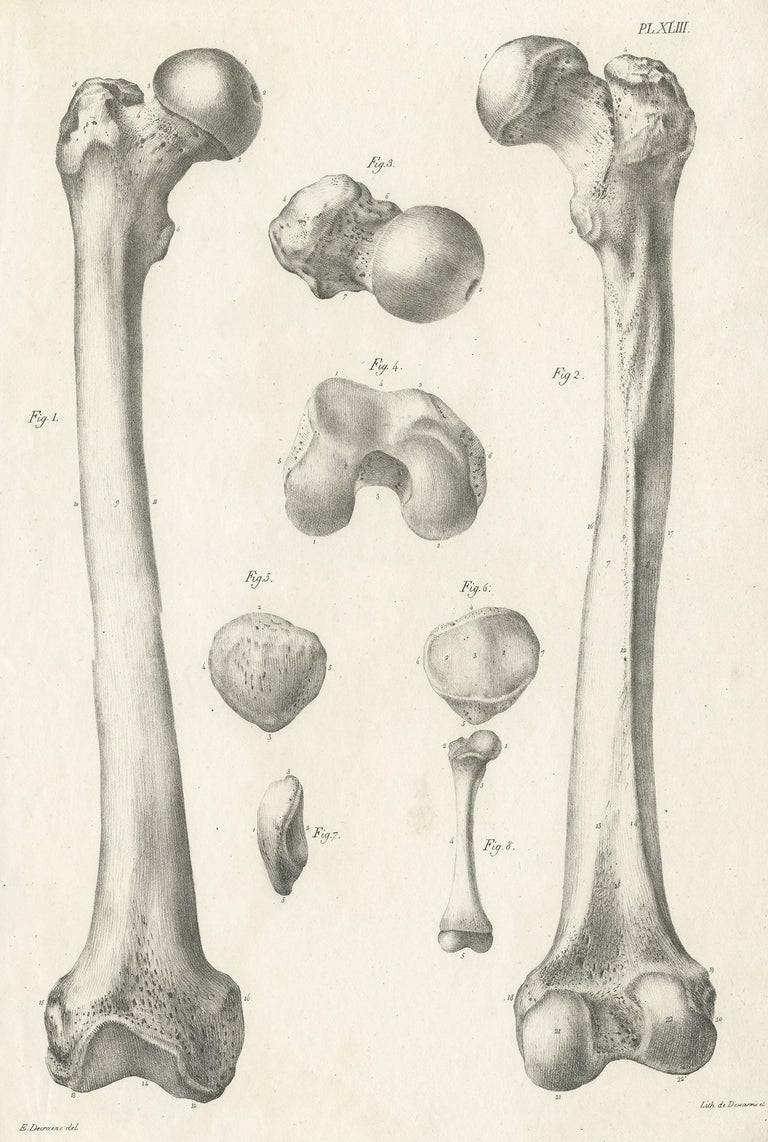The image is a detailed, black-and-white sketch of various human leg bones, resembling an old academic textbook illustration. It features a total of eight distinct bones labeled as fig 1 through fig 8. The illustration is set against an off-white or cream-colored background, adding to its vintage appearance. Dominating the left and right sides of the image are two notably long bones, likely human femurs, characterized by rounded joint structures resembling mushroom tops and typical bone joints at their ends. Interspersed among these large femurs in the center are smaller bones, varying in shape and size. These include a ball joint bone, a half-circle bone with a notch, two circular pieces, an ear-shaped bone, and another straight bone. Additionally, there are cursive annotations in Roman numerals, such as PLXLIII, and smaller, illegible cursive writing at the bottom edges, enhancing the scholarly aesthetic of the diagram.